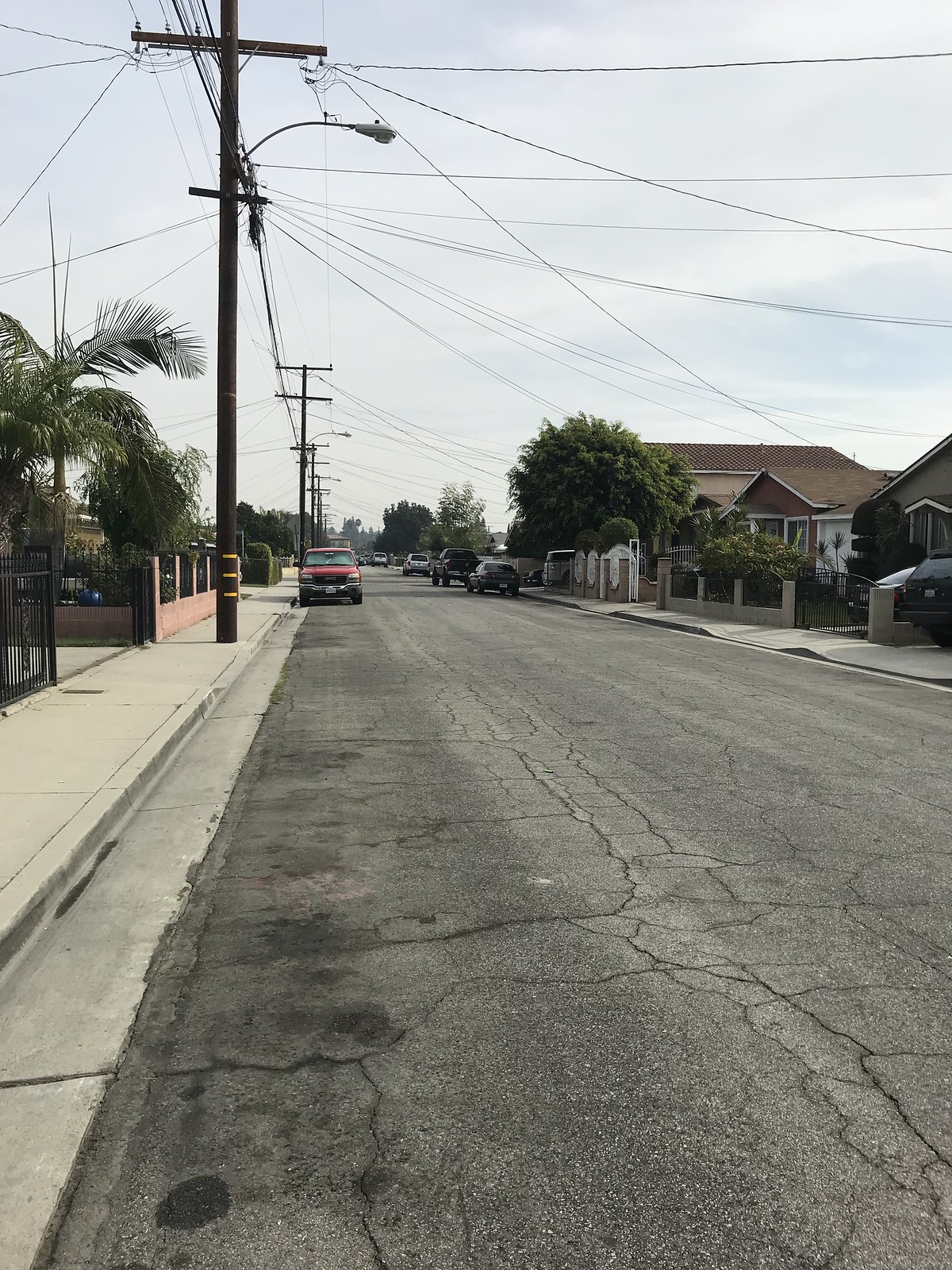The image depicts a typical residential street in the United States, likely situated in a warmer climate, as suggested by the prominent palm tree on the left side of the frame. This could place the location in states such as California, Arizona, Nevada, or Florida. The perspective is from someone looking down the street, which extends for about three blocks.

On the left-hand side, there is a red truck parked near the curb, while the right side of the street hosts about four to five parked cars. This arrangement leaves space for only one car to travel down the street, which would normally accommodate two lanes if not for the parked vehicles. Sidewalks line both sides of the street, bordered by fences that extend to the curb, enclosing residential properties.

Visible on the right are approximately four houses, along with a couple of cars parked in a garage, and some trees providing additional greenery. The street itself shows signs of wear and tear, featuring numerous cracks, darker patches, and oil spills, indicating it has seen better days.

Overall, this is a gray, weathered street in a residential area, complete with the usual landscape of houses, sidewalks, parked cars, and touches of nature.